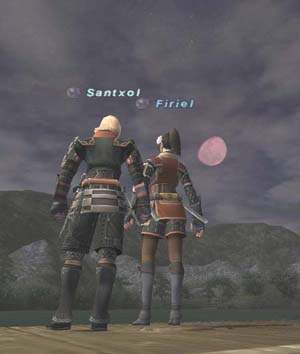Screenshot from the game features two characters, a man and a woman, standing on a wooden platform overlooking a serene water body. The man, positioned on the left, and the woman, on the right, are both clad in full armor. They both appear to have swords sheathed at their sides, ready for battle. Above them, their names are displayed: the man's reads "Sant Oxxel" and the woman's is "Fieryu." In the background, majestic mountains rise toward a sky dotted with white clouds, and a reddish moon can be glimpsed on the far right, adding an ethereal quality to the scene.